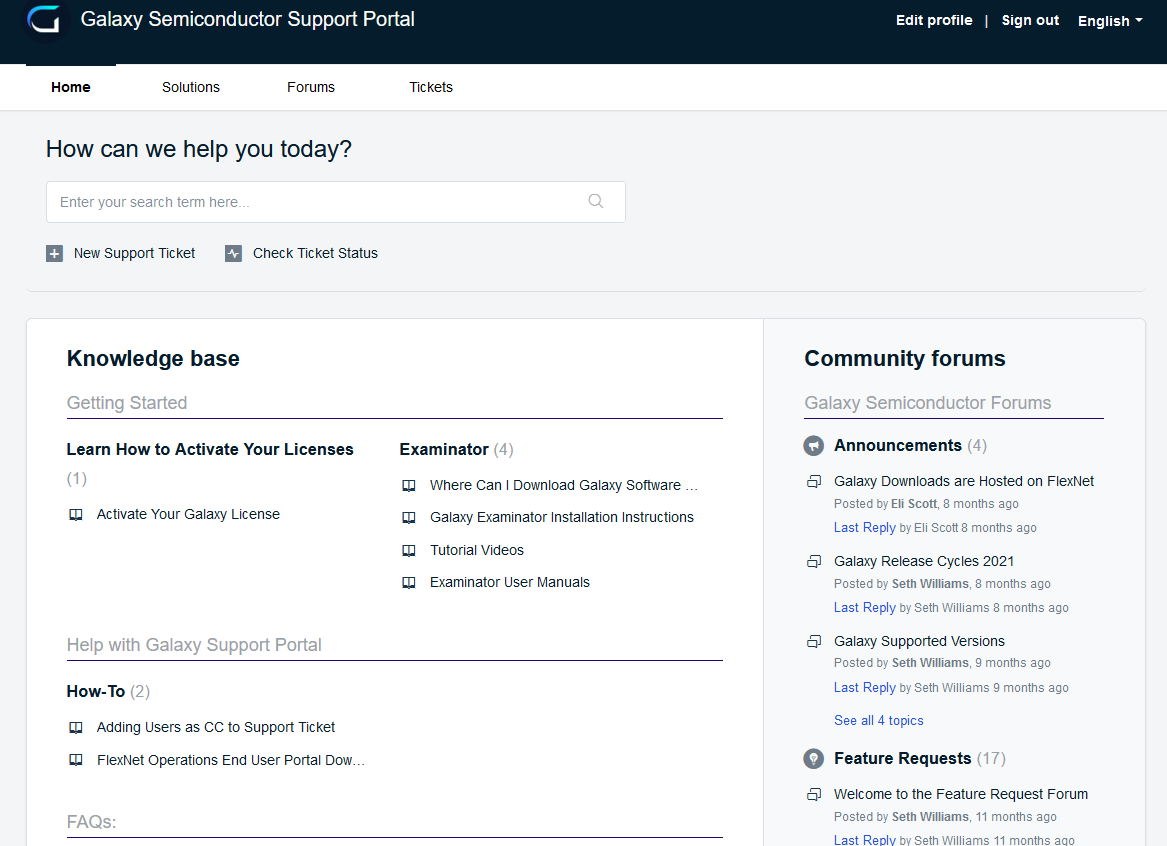**Detailed Website Caption: Galaxy Semiconductor Support Portal Homepage**

The website features a navy blue header with the text "Galaxy Semiconductor Support Portal." The header prominently displays the portal's logo, a stylized blue and white "G" against a blue galaxy background. To the right of the logo, white text options include "Edit Profile," "Sign Out," and "English."

Directly below, a horizontal navigation bar provides easy access to key sections: "Home," "Solutions," "Forums," and "Tickets." Beneath this, a welcoming message reads, "How can we help you today?" followed by an empty search bar that prompts, "Enter your search term here."

Further down, two prominent support options are displayed: "New Support Ticket" with a plus sign icon, and "Check Ticket Status" with a lightning bolt icon. This section is separated from the rest of the content by a horizontal line, all set against a light gray background.

The main content area features several tabs and links for user assistance:
- **Knowledge Base** (black tab)
  - **Getting Started** (section title) followed by a horizontal line
    - **Learn how to activate your licenses** (bold)
      -  **Activate your Galaxy license**: accompanied by a book icon
      -  **Where can I download Galaxy software…**
      -  **Galaxy Examinator installation instructions**
      -  **Tutorial videos**
      -  **Examinator user manuals**
  - **Help with Galaxy Support Portal** followed by a horizontal line
    - **How To** (section title in bold)
      - **Adding users at CC to support ticket** (with book icon)
      - **FlexNet operations in user portal…**

- **FAQs** followed by a horizontal line

- **Community Forums**
  - **Galaxy Semiconductor Forums** followed by a horizontal line
    - **Announcements** (accompanied by a megaphone icon) with "(4)" to its right
      - **Galaxy downloads are hosted on FlexNet**
        - Posted by Eli Scott eight months ago
        - Last reply by Eli Scott eight months ago (in smaller gray text with last reply in blue)
        - Speech bubble icons indicating conversation
    - **Galaxy release cycles 2021**
      - Posted by Seth Williams eight months ago
      - Last reply by Seth Williams eight months ago
    - **Galaxy supported versions**
      - Posted by Seth Williams nine months ago
      - Last reply by Seth Williams nine months ago
      - "See all 4 topics" (blue link text)
  - **Feature Requests** (title in pick poll letters)
    - Light bulb icon
    - "(17)" to the right
    - **Welcome to the feature request form**
      - Posted by Seth Williams 11 months ago
      - Last reply by Seth Williams 11 months ago

This structured and comprehensive overview aids users in navigating various support options and community forums efficiently, ensuring a user-friendly experience.